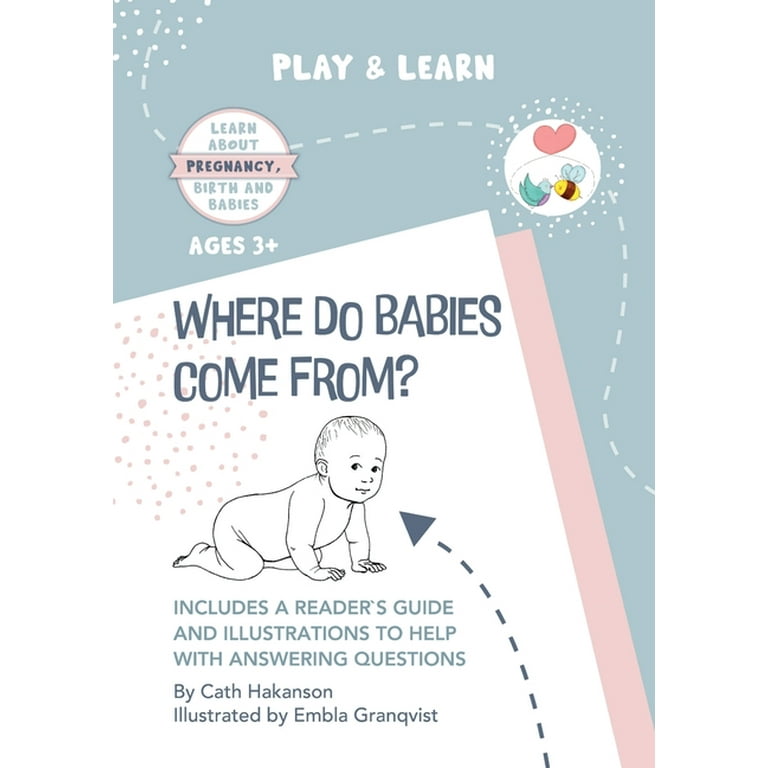The cover of this book, intended to help parents teach children ages 3 and up about pregnancy, birth, and babies, features a vertical rectangular layout with a light bluish-gray background. At the top, white text reads "Play and Learn." Below that, there's a white circle on the left containing the title "Learn About Pregnancy, Birth, and Babies" in blue lettering, accompanied by "Ages 3 plus" in white. A dotted line connects this circle to another white circle on the right, which depicts a bee kissing a bird with a red heart above them. Further down, another section with a white background and a pink border holds the question "Where Do Babies Come From?" in blue lettering. Below this, a line drawing of a crawling baby is shown, followed by the text, "Includes a Reader's Guide and Illustrations to Help with Answering Questions." The book is authored by Kath Hakanson and illustrated by Embla Granquist, with an arrow pointing from the baby image upward. The overall design, with its playful and informative visual elements, aims to engage young children in learning about the origins of babies.